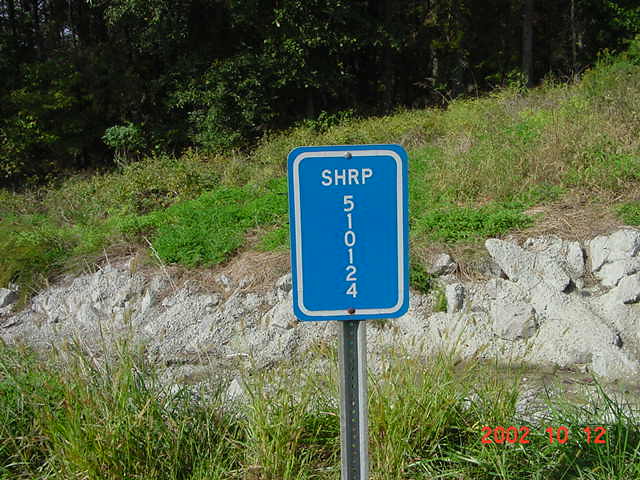In the photograph, a small rectangular sign, mounted on a lone grey metal pole, stands amidst nature's embrace. Behind it, a dense forest teems with trees, their leafy canopies forming a verdant backdrop. Closer to the sign, sporadic tufts of grass and resilient weeds pepper the ground, thriving even as they cling to the rugged rock face that rises just behind the sign.

The sign itself, approximately a foot tall and three-quarters of a foot wide, features a vivid blue background bordered by a white stripe. Central to the rectangular sign, the bold white font reads "S-H-R-P," followed by the consecutive numbers "5-1-0-1-2-4" below. At the bottom right corner of the image, a time stamp in bright orange denotes the date: "2002-10-12," adding a historical touch to this serene slice of nature captured forever in a photograph.